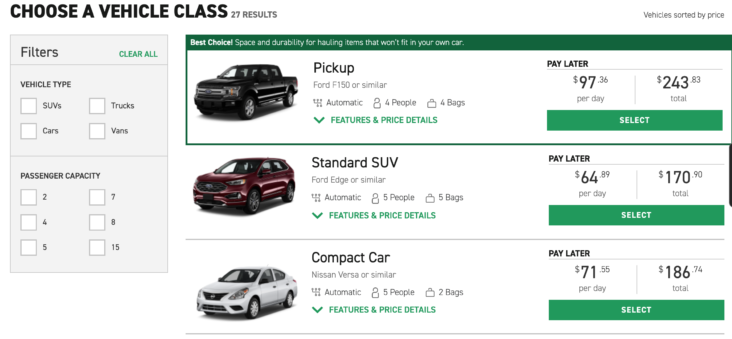The image depicts a horizontally oriented screenshot of a car rental agency website. At the top left corner, large black text reads "Choose a Vehicle Class," indicating that there are 27 available results. A light gray filters box is positioned on the left side of the page.

Directly below the "Choose a Vehicle Class" heading, users can filter their vehicle selection by types such as SUVs, cars, trucks, and vans, as well as by passenger capacity options of 2, 4, 5, 7, 8, or 15 passengers. The top section is highlighted with a green outline, featuring a horizontal box that contains a photograph of a black pickup truck. A green banner above this photo proclaims it as the "Best Choice for Space and Durability for Hauling Items That Won't Fit in Your Own Car."

The top right corner of the page indicates that the vehicles are sorted by price. The black pickup truck, available for a pay-later rate, costs $97.36 per day with a total rental cost of $243.83. A green "Select" button is positioned below this information.

Also displayed are two other vehicle options: a red standard SUV priced at $64.89 per day and a white compact car available for $71.55 per day.